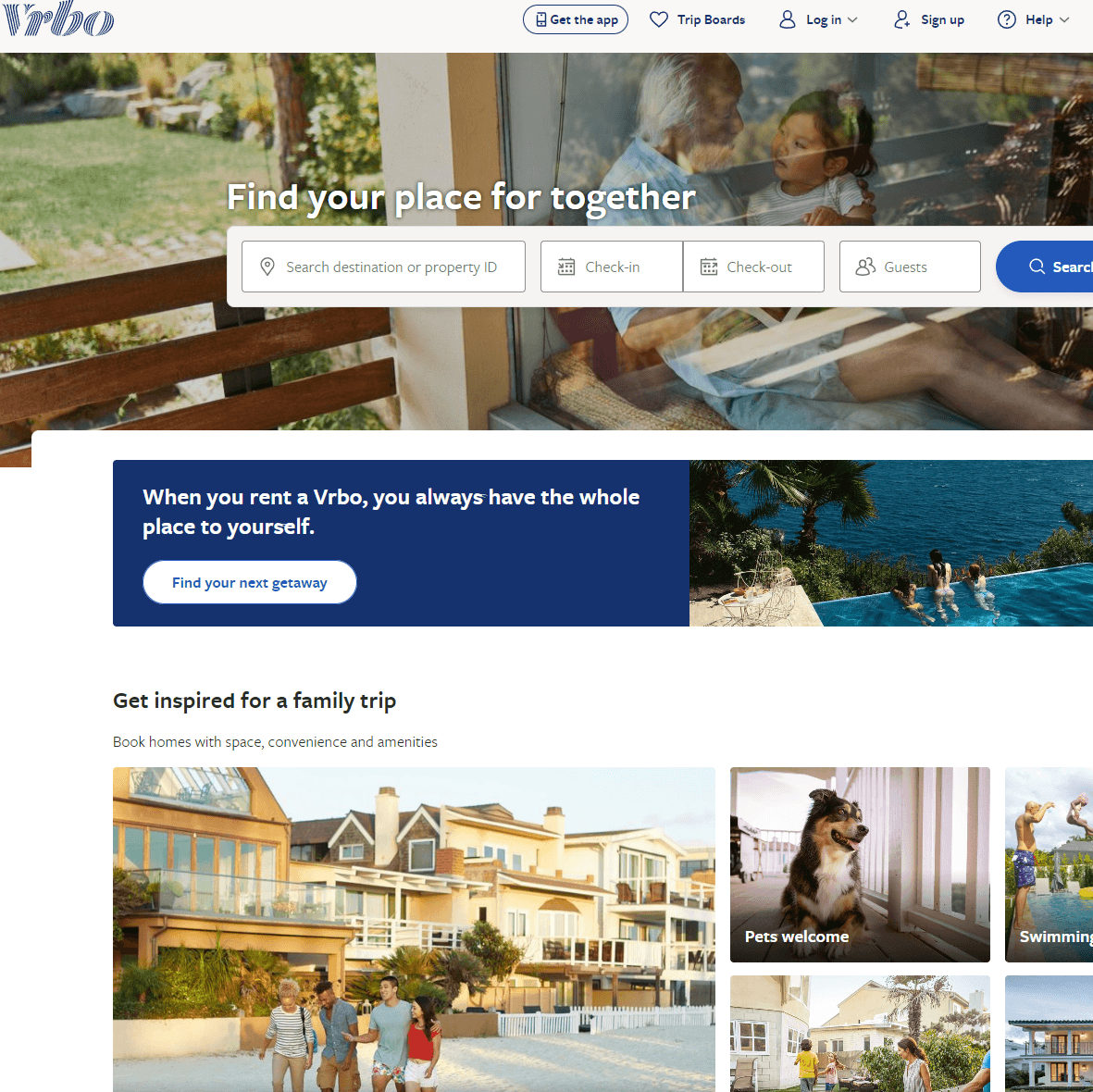Screenshot featuring a white background with various elements highlighting VRBO services and functionalities. At the top, navigation options include "Trip Boards," "Log In," "Sign Up," and "Help." 

The primary banner showcases a heartwarming image of a granddad with his grandson, with the tagline "Find Your Place for Together." Below this, there's a comprehensive search bar featuring fields for "Check-in," "Check-out," "Guests," and a blue oval button with a white magnifying glass labeled "Search."

Highlighted content sections include:
1. A photograph of three people enjoying a pool near the beach with the statement: "When you rent at VRBO, you always have the whole place to yourself. Find your next getaway." 
2. An inspiration section showing teens walking with urban buildings in the background, captioned: "Get inspired for a family trip. Book homes with space, convenience, and amenities."
3. A welcoming note for pet owners accompanied by a picture of a dog and the label "Pets Welcome."
4. Various images depicting vacation scenarios, including swimming and people strolling through town.

The interface is designed to encourage users to explore and book family-friendly vacation homes with ample space and amenities.